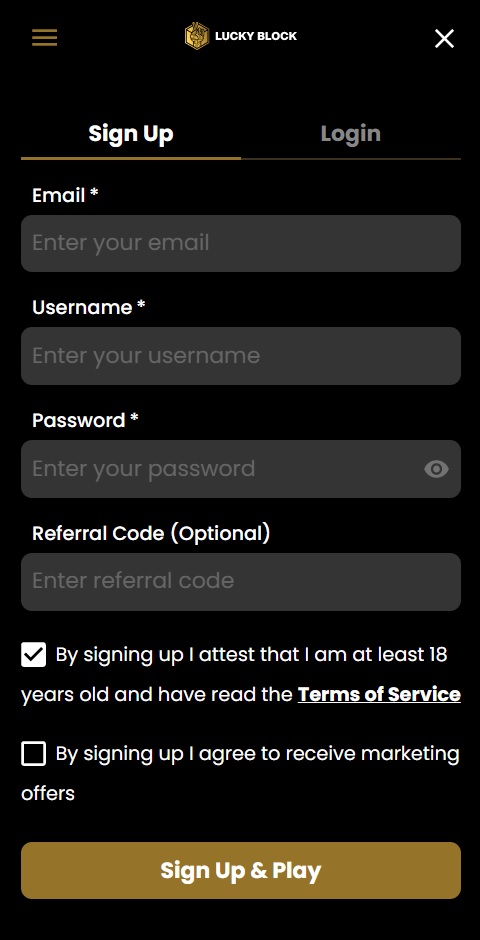**Caption:**

The image depicts a detailed screenshot of the sign-up page for "LUCKY BLOCK," prominently displayed in bold capital letters at the top. In the upper right corner, there's a small "X" button, while the top left corner features a golden icon with three horizontal lines. Below the title, the page offers two primary actions: "Sign Up" and "Log In."

The first field asks for an email address, followed by a section labeled "Username," indicated with an asterisk (*) to denote it as a required field. The adjacent input box prompts the user to "enter your username." Next, the "Password" field is similarly marked with an asterisk and instructs users to "enter your password," ensuring secure data entry with starred characters.

An optional "Referral Code" field follows, where users can input a referral code if they have one. Below this, there is an already-checked checkbox stating: "By signing up, I attest that I am at least 18 years old and have read the Terms of Service," with "Terms of Service" being a clickable hyperlink. Another checkbox, left unchecked, gives users the option to agree to receive marketing offers.

At the bottom of the form is a prominent gold and white "Sign Up and Play" button, inviting users to complete their registration and start engaging with the platform.